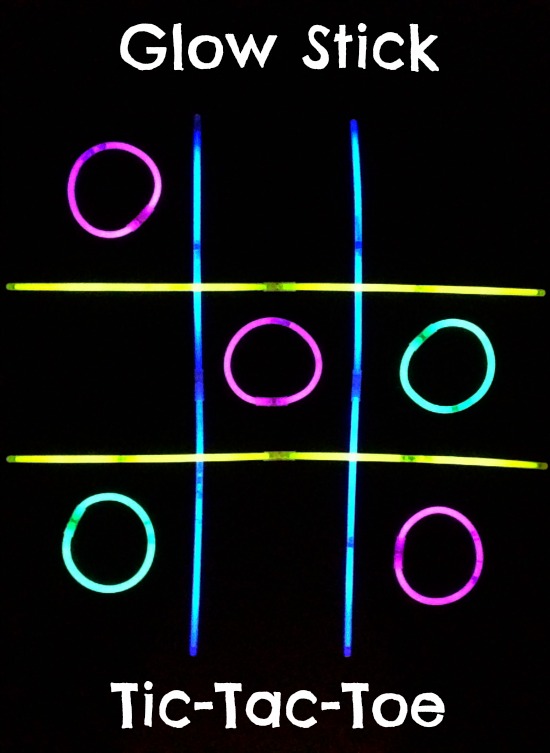This black and white image features a glowing neon tic-tac-toe game. The word "Glowstick" is prominently displayed at the top in white font, while "Tic Tac Toe" is written in white at the bottom. The black background is contrasted by a vibrant tic-tac-toe grid, with two vertical neon blue lines and two horizontal neon yellow lines intersecting in the middle. The game contains a total of five circles, all in neon colors. Three pink circles form a winning diagonal line from the top left to the bottom right. The remaining two circles, colored light green, are positioned in the bottom left and middle right, appearing to have lost. The dynamic neon colors create a vivid contrast against the solid black background, highlighting the overall "glowstick" theme.